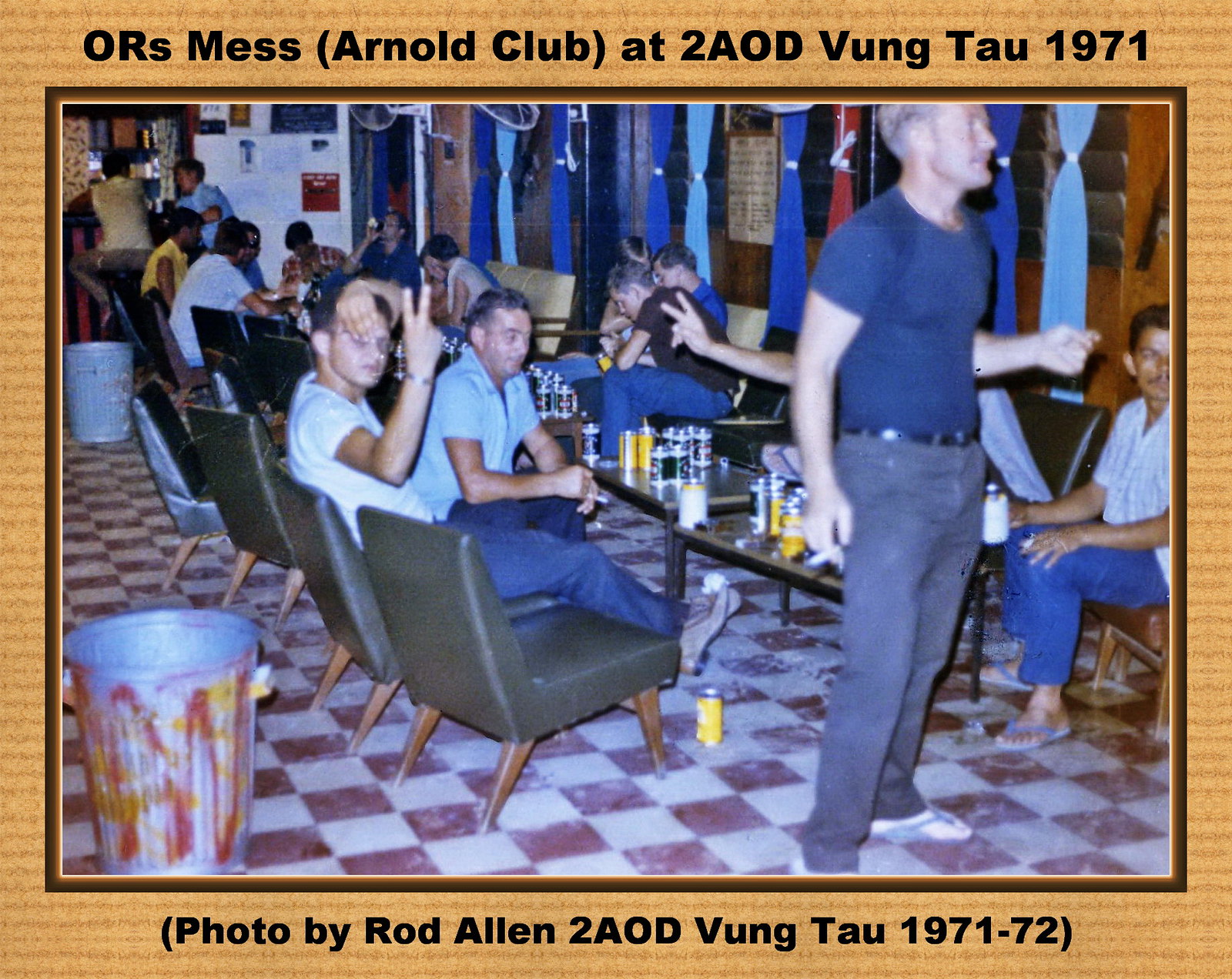The image captures a lively scene in what appears to be a nostalgic bar or restaurant setting with a checkered red and white tile floor. The photograph, bordered in light orange, prominently features black text at the top that reads, "ORS Mess (Arnold's Club) at 2AOD Vung Tau 1971," and below it, in parentheses, "photo by Rod Allen, 2AOD Vung Tau 1971-72."

Several men in short-sleeved shirts are scattered throughout the indoor space, either sitting on gray leather seats or standing. A man on the left in a white shirt holds up a peace sign, while another man to the right, dressed in a blue shirt and gray pants, stands nearby. The tables in front of them are cluttered with numerous drink cans, likely beer, indicating a casual, party-like atmosphere. In the background, there are tin trash cans behind the chairs, adding to the old-school charm of the place. Most of the men are preoccupied with drinking and chatting, with only a couple acknowledging the camera.